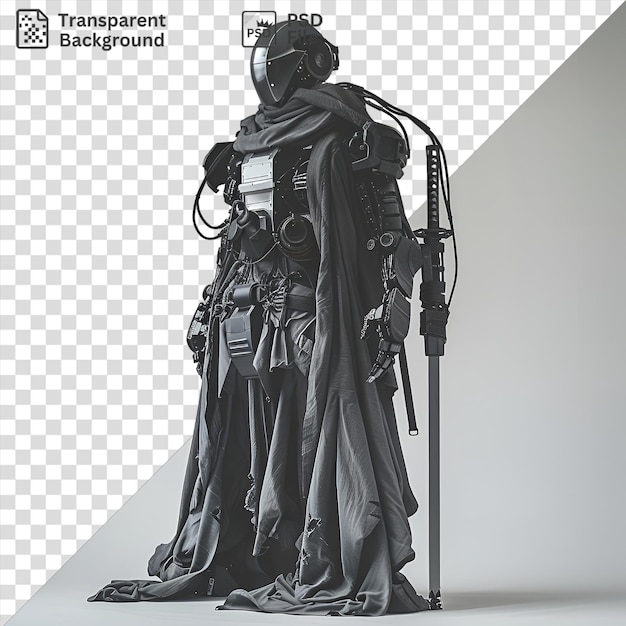The image is a digitally created advertisement by Photoshop showcasing a futuristic, black and white Star Wars-like character. The character stands at the center, adorned with a smooth black helmet featuring a reflective visor that conceals the face, and a cloth scarf that cascades down, pooling at the ground. His right arm appears robotic, and he has a sword or lightsaber attached to his back. From his neck, cords run to the sword and to his arms, enhancing his cyborg appearance.

The background is divided diagonally. The top left segment displays a gray and white checkerboard pattern with "transparent background" written in the corner, signifying a transparent section once exported. The letters "PSD FIL" also appear, accompanied by a PSD logo crowned over the letters. The bottom right segment retains a light gray background, contrasting with the transparent section and emphasizing the meticulously detailed character.